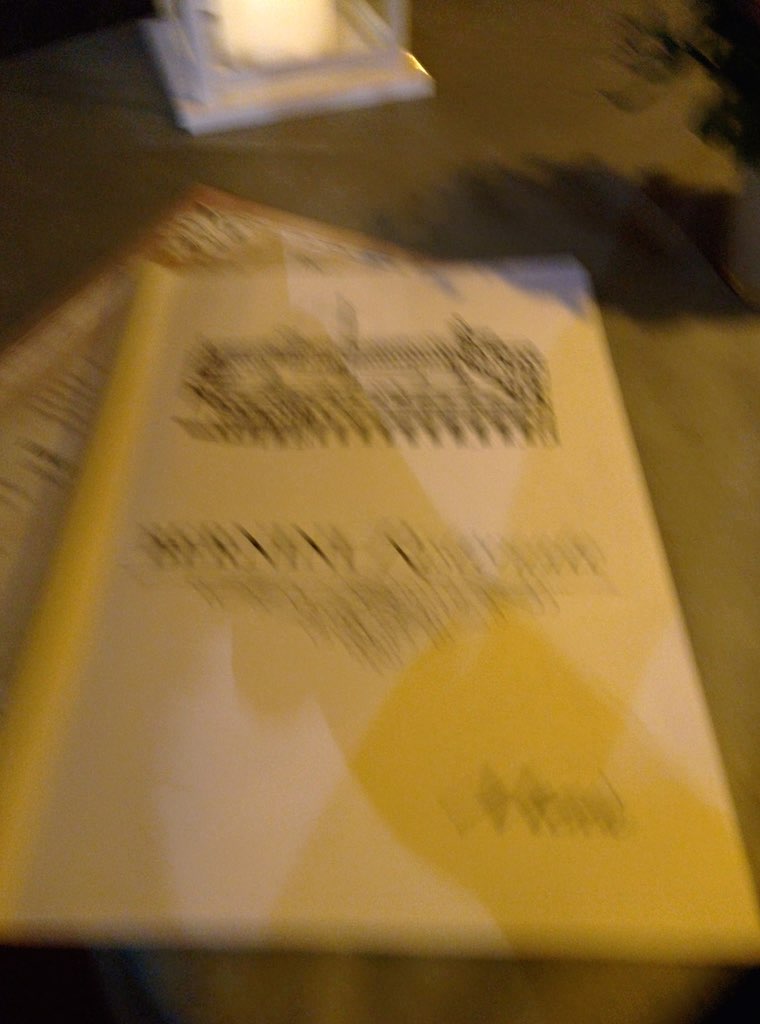The photograph is very blurry, making it difficult to discern fine details. However, it appears to depict a rectangular menu or a pamphlet with a white background and a yellow border along the left side, placed on a brown table. The top of the menu features a brown rectangle with some designs that are indistinguishable due to the blurriness. Below this rectangle, there is black writing in the center. To the upper left of the photo, a white square base with what might be a white candle can be seen, suggesting it could be part of a table centerpiece. Additionally, towards the top right of the image, the presence of a plant is noted, possibly another part of the table decor. Below the menu, there seems to be another piece of paper, partially visible. The photograph also shows a shadow cast, likely from another object on the table.